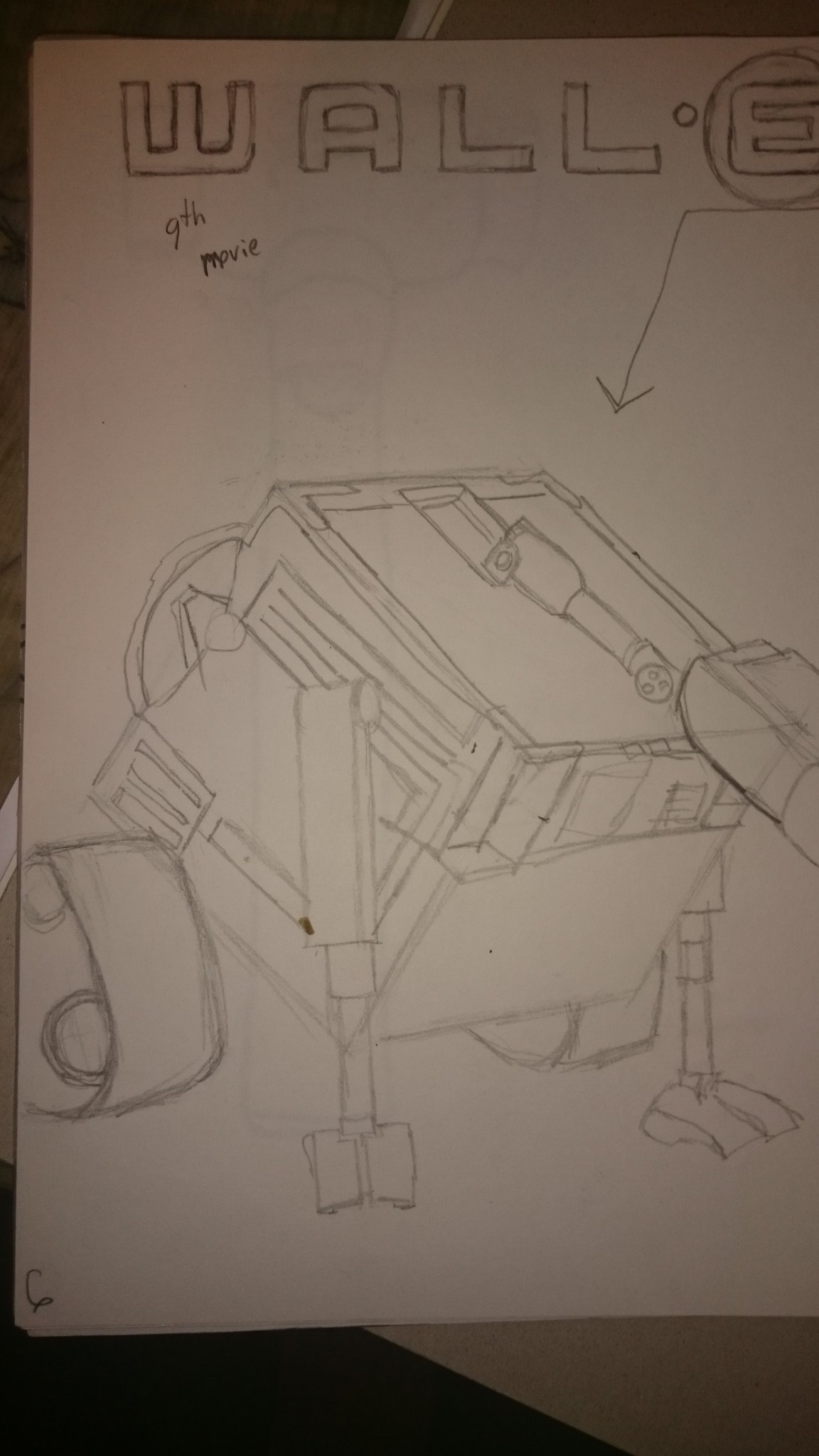This detailed caption describes an intricate black ink drawing on a piece of white paper. At the top center of the drawing, the word "WALL" is prominently written. In the top right corner, there's a circled letter "E." Below this, the phrase "9th MOVIE" is inscribed. An arrow descends from the top right, directing attention to a machine illustrated beneath it. The machine has a square-shaped body and is equipped with wheels on either side. Extending from the sides of the machine are limbs, which could be interpreted as either legs or hands, ending in flat tips. Additionally, there's a protrusion emerging from the top of the machine, adding to its complexity.